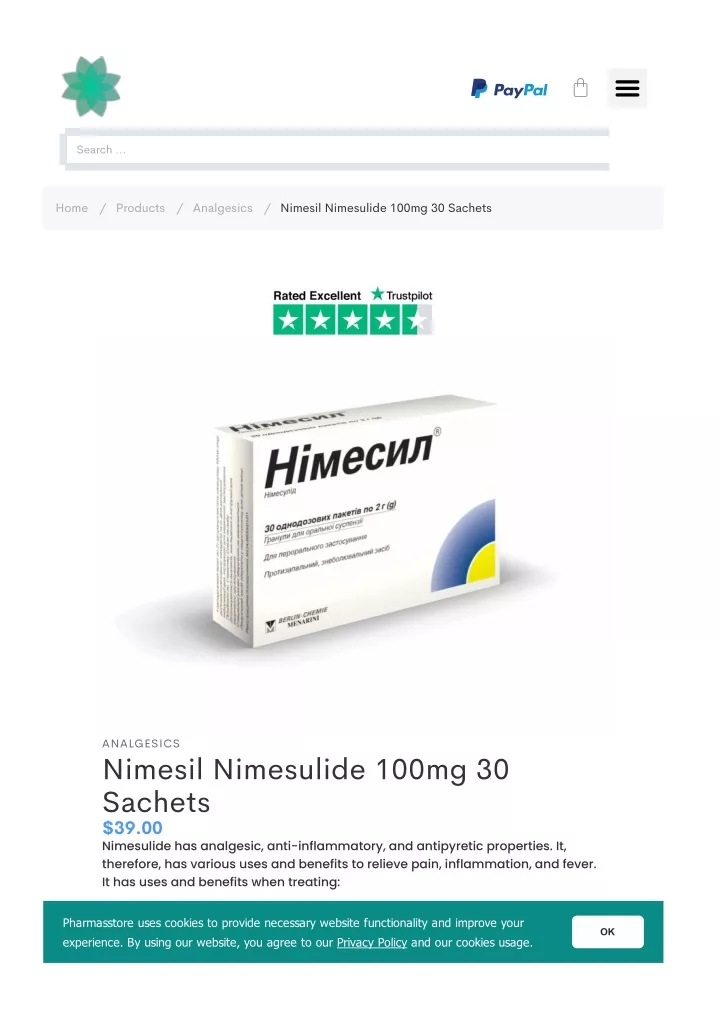The image appears to be an online advertisement or webpage showcasing a medication product. In the upper left corner, there is a simple, cartoonish sun icon against a light green background. Moving to the right, the PayPal logo is prominently displayed, indicating the availability of a payment method. Next to this, there are navigational bars for various sections of the site, including Home and Products.

The featured product is an analgesic called "Nimial Nilcide." Specifically, it is a 100-milligram dose available in a box containing 30 sachets. The box has a rectangular cube shape, and in the bottom right corner, there is a partial circular design – the outer part of which is blue, transitioning to yellow near the corner. The circle is inscribed with the product details: "Analgesics, Nimicil, Nimacilidide, 100 milligrams, 30 sachets." This medication appears to be an anti-inflammatory aimed at relieving pain, inflammation, and fever.